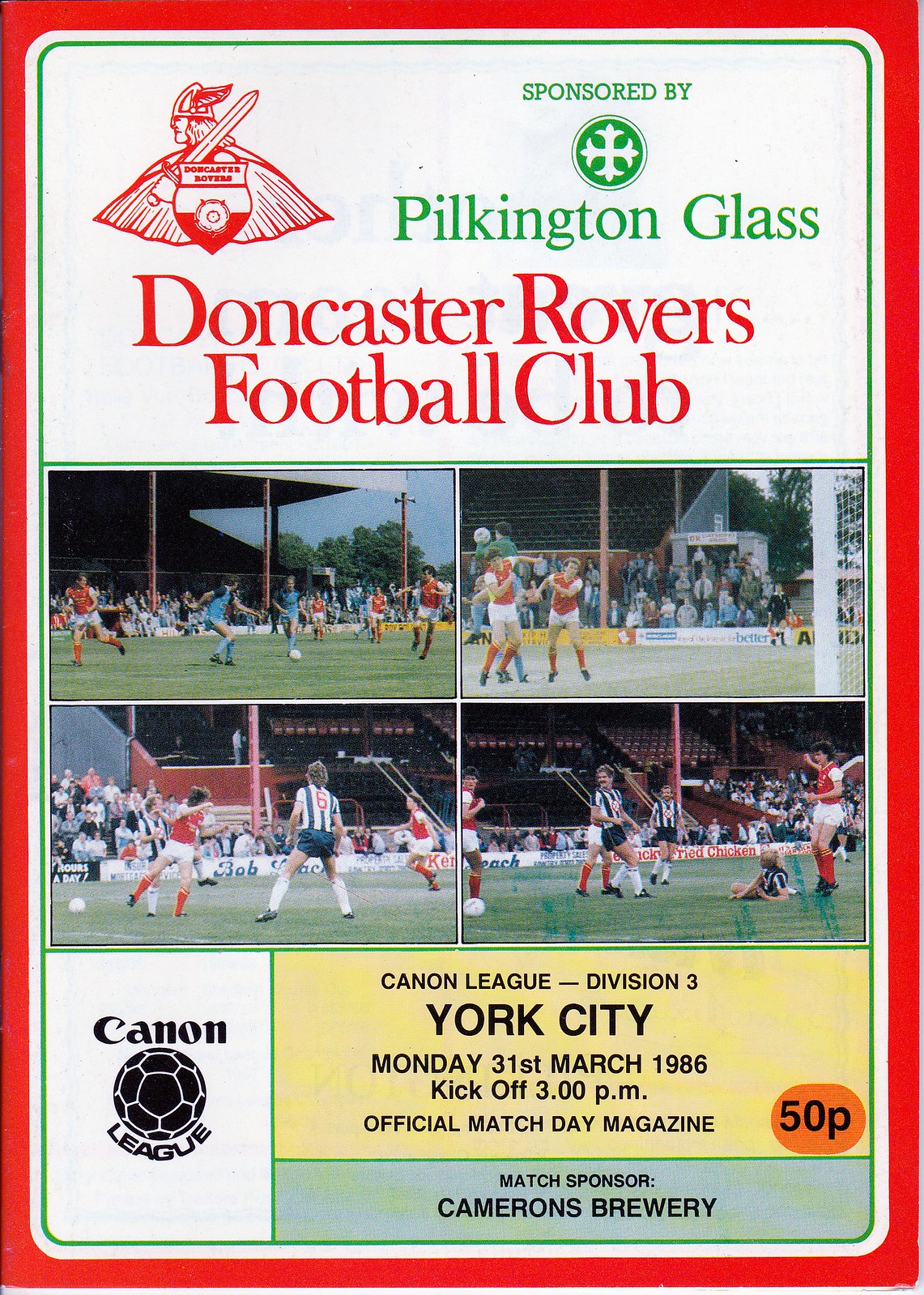**Caption:**

A vintage flyer for the Doncaster Rovers Football Club, promoting a match in the New York City league division. The kickoff is scheduled for Monday, March 31st, 1986, at 3:00 PM. The flyer, possibly the cover of a magazine, is sponsored by Cameron's Brewery and Pilkington Glass. The design features an eye-catching bright red outline with accents of green and yellow, indicative of its age. In the middle section, there are four action-packed images of soccer matches, showcasing players in their iconic red tops and white shorts.